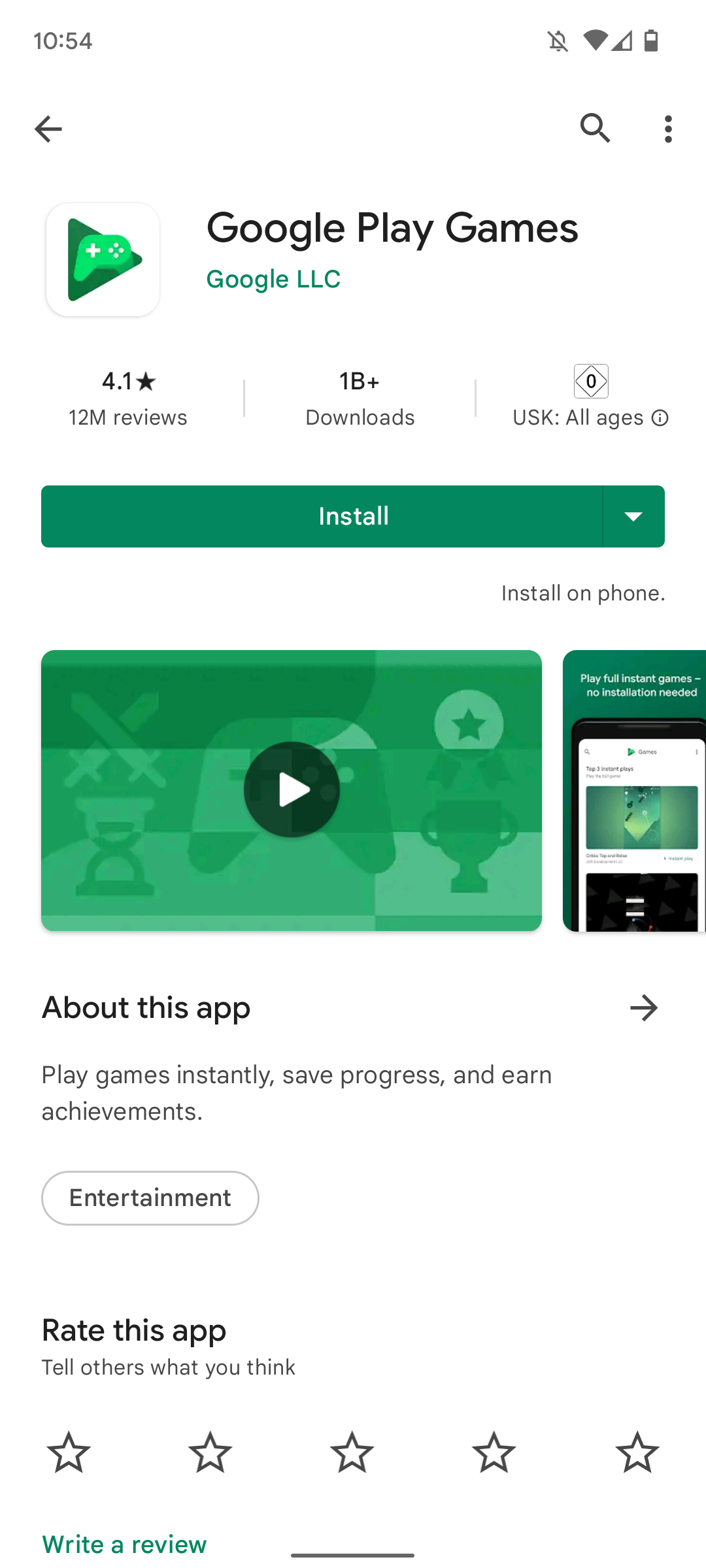A detailed screenshot from a mobile device showcases the Google Play Games page within an app store. At the top of the device's interface, the time is displayed on the left as 10:52, accompanied by icons on the right indicating muted notifications, Wi-Fi signal, data strength, and a battery level slightly over halfway. 

The app in focus is Google Play Games, developed by Google LLC. The app's icon—a green controller within a red play button—and its title are placed prominently at the top. It boasts a 4.1-star rating based on 12 million reviews, with over 1 billion downloads and a USK rating for all ages. 

Directly below, a green "Install" button is visible, followed by an "Install on phone" label. Information about the app is presented further down, including a playable thumbnail with a green overlay featuring symbols of a gaming controller, hourglass, crossed swords, and a trophy. To the right of this thumbnail, a screenshot is also displayed.

The bottom section of the screenshot reads "About this app," followed by phrases like "Play games instantly, save progress, and earn achievements." Categorized under "Entertainment," users are prompted to rate the app, with a five-star rating system and an option to "Write a review."